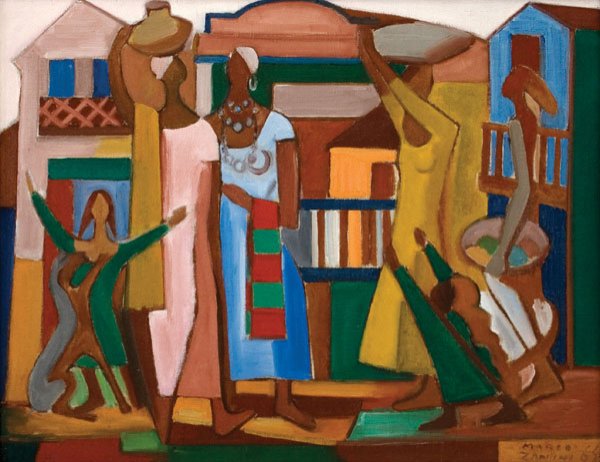This vibrant, modern art painting depicts a dynamic cityscape featuring African women engaged in their daily activities. The background is filled with colorful buildings in shades of beige, green, yellow, and dark blue, each detailed with fences, banisters, and windows. The ground appears to be a mosaic of multicolored tiles. On the left side of the painting stands a light brown-skinned girl with short brown hair, clad in a green dress, her hands outstretched upwards. Next to her, an adult woman with a headscarf wears a long light pink short-sleeved shirt and balances a pottery piece on her head. Beside her is another woman in a blue dress adorned with jewelry and earrings, also holding a basket on her head. Further to the right, a woman dressed in a long-sleeved yellow dress carries a basket and is approached by a small child in a dark green dress with arms outstretched. On the far right, a tall, thin woman in a long brown dress carries a basket. The overall scene is rich with shades of brown, tan, blue, green, red, pink, and hints of orange, capturing the essence of a vibrant African community. The artist's signature, a scrawled MZ, is visible in the lower right-hand corner, suggesting authenticity and a subtle personal touch.